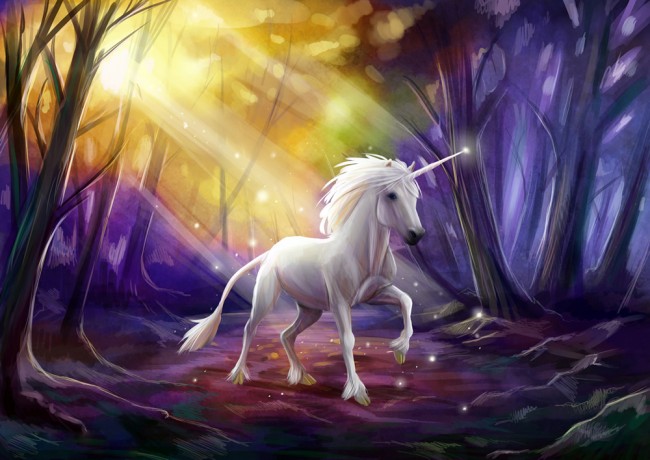In this captivating digitized painting, a majestic white unicorn with a shimmering white mane and classic horn stands gracefully amidst a mystical forest. Its dark, expressive eyes and black nose add a touch of contrast, while its raised right leg gives the impression of a gentle, poised walk. The unicorn appears to be subtly moving to the right but also facing forward slightly, under the enchanting glow of sunlight that streams through the treetops from the top left. This light casts a golden hue on the left side of the forest, contrasting dramatically with the deep purples and blues that dominate the scene. The trees, devoid of leaves, lend an otherworldly feeling, with sparkles and floating white particles adding to the ethereal ambiance. The forest floor transitions from dark purples and blacks to lighter shades, enhancing the enchanting atmosphere of this sci-fi-like depiction. The overall scene is vibrant yet dark, with a mystical and surreal quality that would make for an enthralling desktop wallpaper.